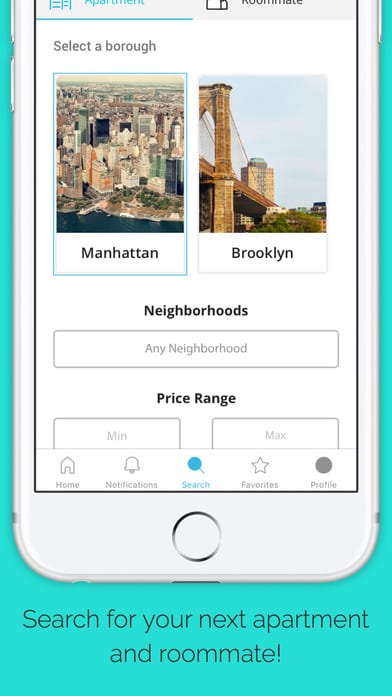The image is a photograph of a white smartphone displaying an apartment search interface. The background is teal, matching the interface's dominant color scheme. At the very bottom of the screen, the text "Search for your next apartment and roommate" in thin black font is visible. The phone itself shows a home button, a circle at the bottom center, and features two side buttons on the top left and one on the top right.

In the interface displayed on the phone, there are two teal-colored categories near the top: "Apartment" and "Roommate," with "Apartment" being currently selected. Below this, the text "Select a Borough" appears, accompanied by two options: "Manhattan" on the left and "Brooklyn" on the right. Manhattan, selected, is marked with a teal border and has an image of the city above it.

Further down, the word "Neighborhoods" appears, followed by a selection box labeled "Any Neighborhood." Below this, the text "Price Range" is displayed, with two boxes beneath it for "Min" and "Max" price entries. At the very bottom of the phone's interface are several icons representing different functionalities: Home, Notifications, Search, Favorites, and Profile.